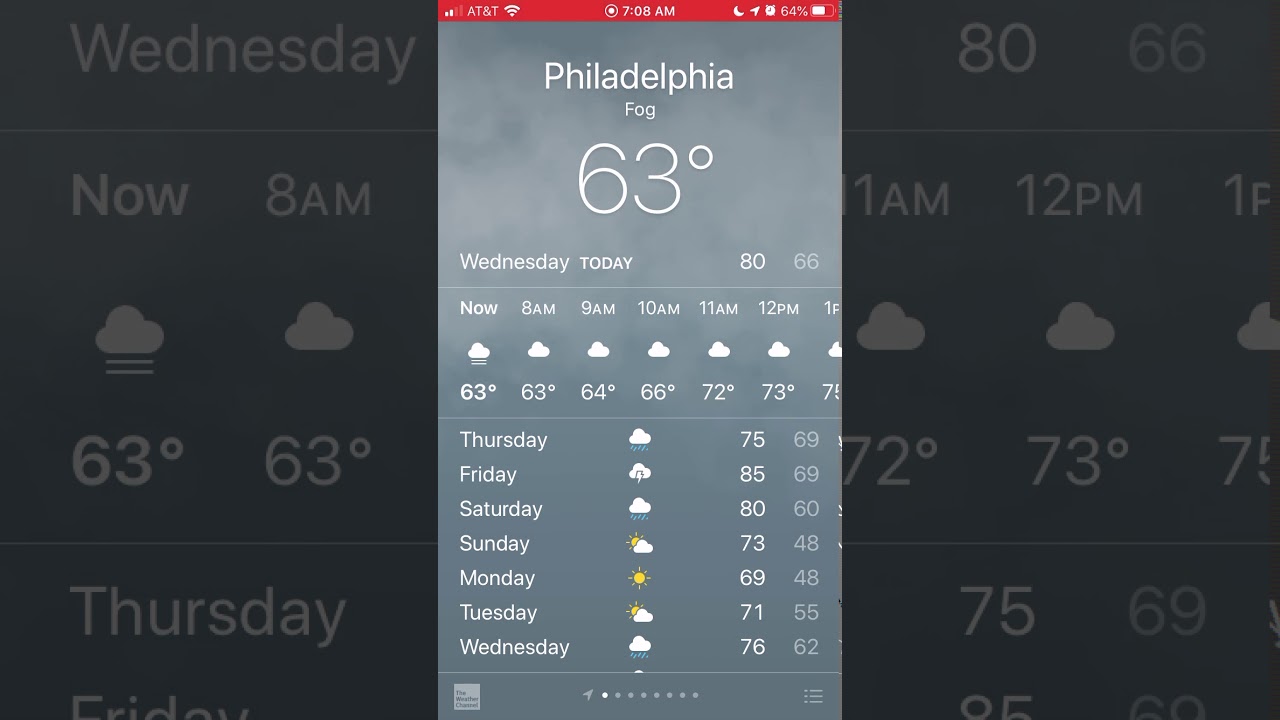This screenshot captures the weather forecast from a mobile app, focusing specifically on the city of Philadelphia. The main application background presents the detailed weather forecast for Wednesday at various times of the day: 'Now,' 8 a.m., 11 a.m., 12 p.m., and 1 p.m. Each time slot is accompanied by an icon depicting the expected sky conditions, along with the corresponding temperature. The display includes multiple days' forecasts arranged vertically across the page.

A secondary overlay box at the forefront highlights Philadelphia's weather details. At the top of this box, a red banner displays the AT&T network information, the current time of 7:08 a.m., and standard mobile status icons such as the battery level and signal strength. Directly below the city name "Philadelphia," the forecast for Wednesday is prominently featured, followed by predictions for the upcoming days extending through to the next Wednesday. This detailed and organized layout offers a comprehensive view of Philadelphia's weather patterns for the upcoming week.